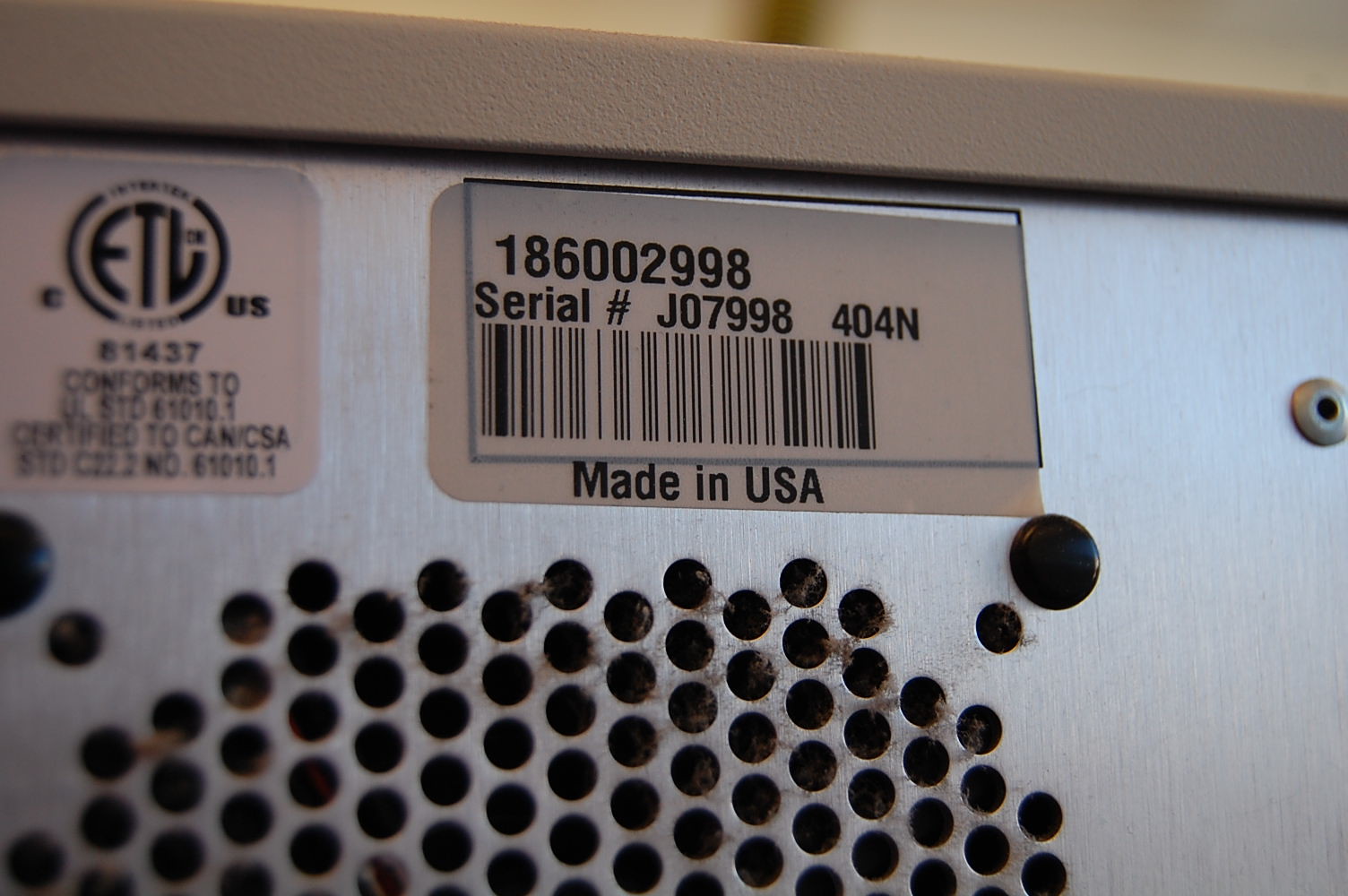A close-up image reveals the rear view of a computer, highlighting intricate details. The top portion features a distinct, grayish metallic frame that lends structural support. At the top-right corner, a small section of the background is visible, albeit blurred and narrowing towards the left. Positioned just below the upper middle of the computer's back are two notable stickers: a serial number UPC code and a white square label to its left. Beneath these identifiers are circular ventilation cutouts designed to enhance airflow and maintain optimal internal temperatures.